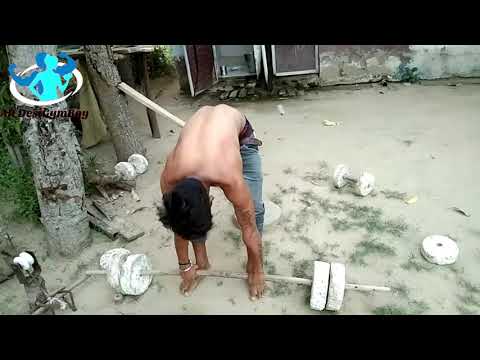In this rectangular image, there are black strips bordering the top and bottom. In the top left corner of the actual picture, there is a logo featuring turquoise and blue silhouettes of two people encircled by a yellow ring, with some lettering beneath it. The picture depicts a man outdoors on a dirt ground, heavily bending over towards the viewer, which obscures his face. He has black hair, no shirt, and is wearing low, raggedy blue jeans that reveal dark underwear. His feet are bare as he arches his back in a problematic way while holding onto a makeshift barbell—a stick with round stone discs on each end. Behind him, similar homemade dumbbells with shorter sticks and stone weights are scattered around. The background includes the bases of trees and a building. The overall color scheme is dull green and gray, making the man’s figure the brightest element in the image.